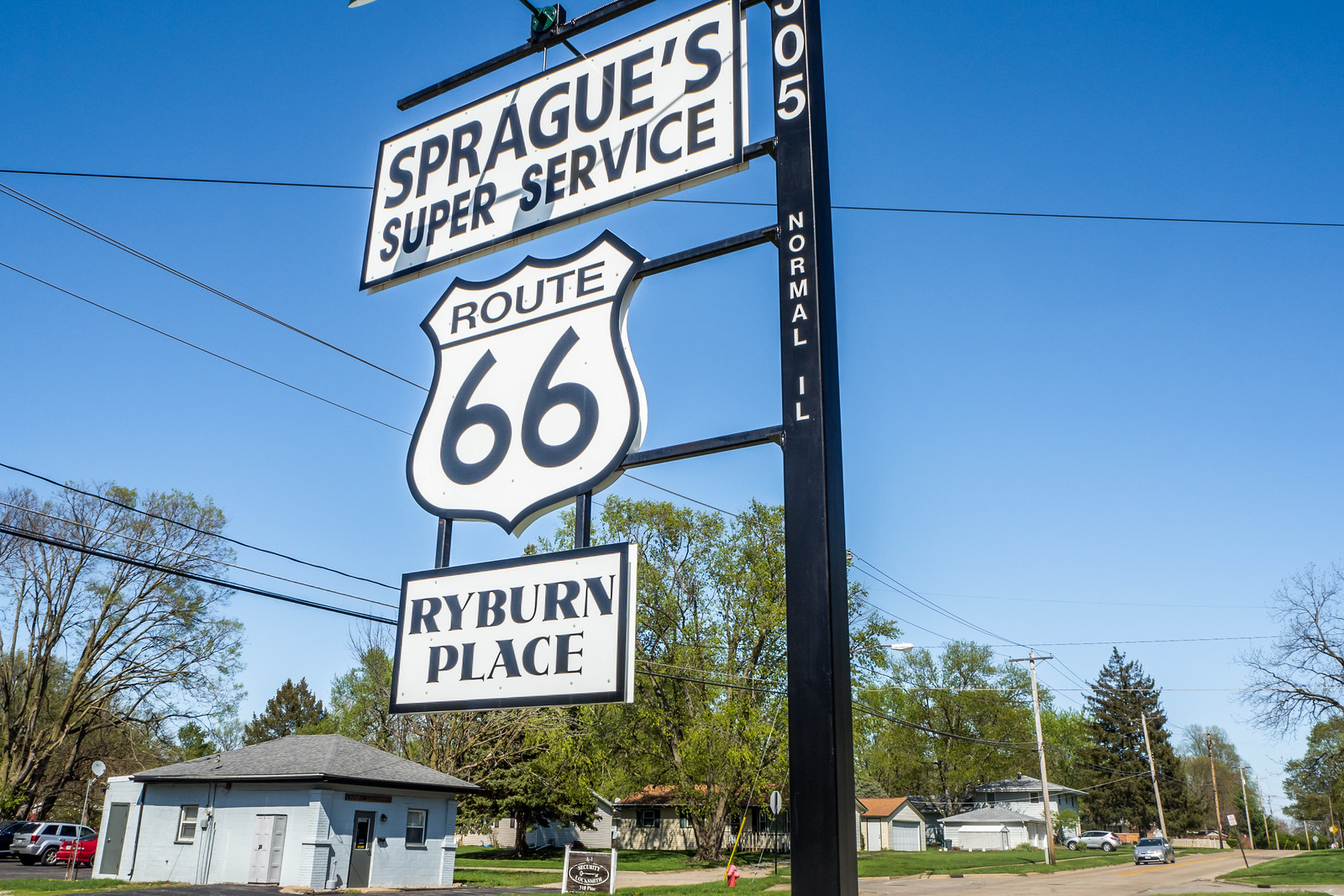This photograph captures a detailed scene of a signboard erected on the side of a road in a neighborhood during a clear, cloudless day. The signboard, firmly attached to a tall, black, squared metal pole, features three distinct sections with text in dark blue against a white background. The topmost section reads "Sprague Super Service," followed by a "Route 66" sign in the middle, and "Ryburn Place" at the bottom. This pole is prominently centered in the image and is accompanied by horizontal bars extending to support the signs.

Surrounding the signboard, the scene includes a road with a car driving towards the viewer, houses, trees, grass-covered ground, and a stone structure resembling a small park facility, complete with outdoor bathrooms, in the lower left-hand corner. Additional cars are parked nearby, and power lines stretch across the neighborhood. The sky is a deep blue gradient, becoming lighter closer to the horizon, and is entirely free of clouds, enhancing the brightness and clarity of the landscape.